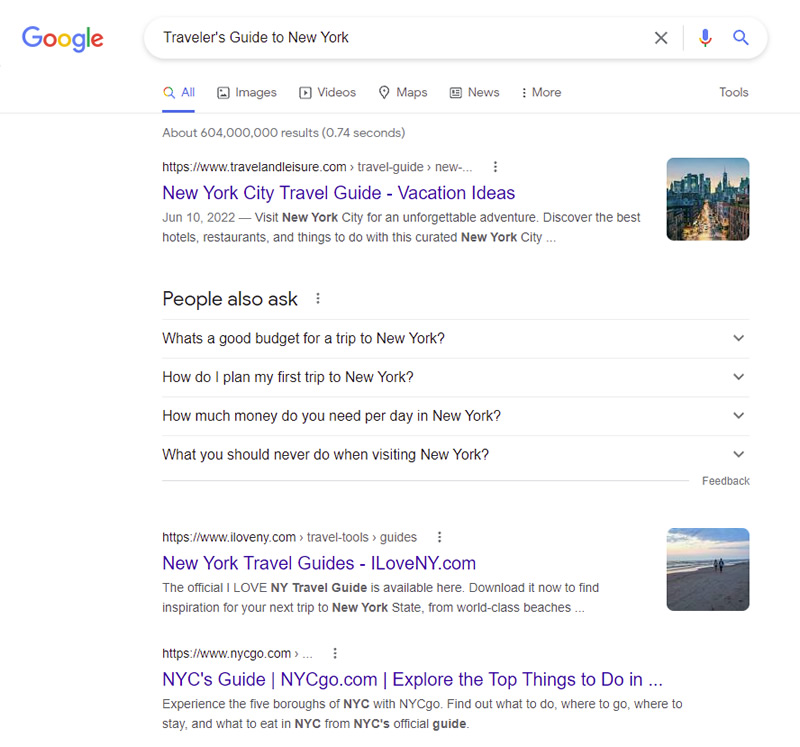The screenshot depicts a Google search results page, illustrating a query for "Traveler's Guide to New York." 

At the top left, the Google logo is clearly visible in its traditional colors: a blue uppercase 'G,' followed by a red 'o,' a yellow 'o,' a blue 'g,' a green 'l,' and a red 'e'. Adjacent to the logo on the right is an elongated search bar where "Traveler's Guide to New York" is typed in black lettering. To the right of this text within the search bar, there is a gray 'X', followed by a thin gray vertical divider line. Further right, the search bar features a microphone icon in Google's signature colors, and to the immediate right of this is a blue magnifying glass symbolizing the search function.

Right below the search bar is a navigational menu. The tab labeled "All" is actively selected, distinguished by its bold blue underline and blue text. The subsequent options—"Images," "Videos," "Maps," "News," and a "More" dropdown menu signified by three dots—are displayed in gray text. To the far right of this menu, "Tools" is also written in gray. A faint, light gray line delineates the menu from the search results below.

Underneath the menu, a light gray line informs that there are "About 604,000,000 results (0.74 seconds)." Following this, the listing of search results begins. The first link, showcased in black text, reads "https://www.travelandleisure.com" with a gray arrowhead pointing to the right. The clickable header of this result is highlighted in blue and reads "New York City Travel Guide – Vacation Ideas," flanked by a dash. Next to this text on the right, a small image depicts a cityscape with a blue sky transitioning to a yellow hue.

This detailed description encapsulates the elements and layout of the Google search results page for the specified query.